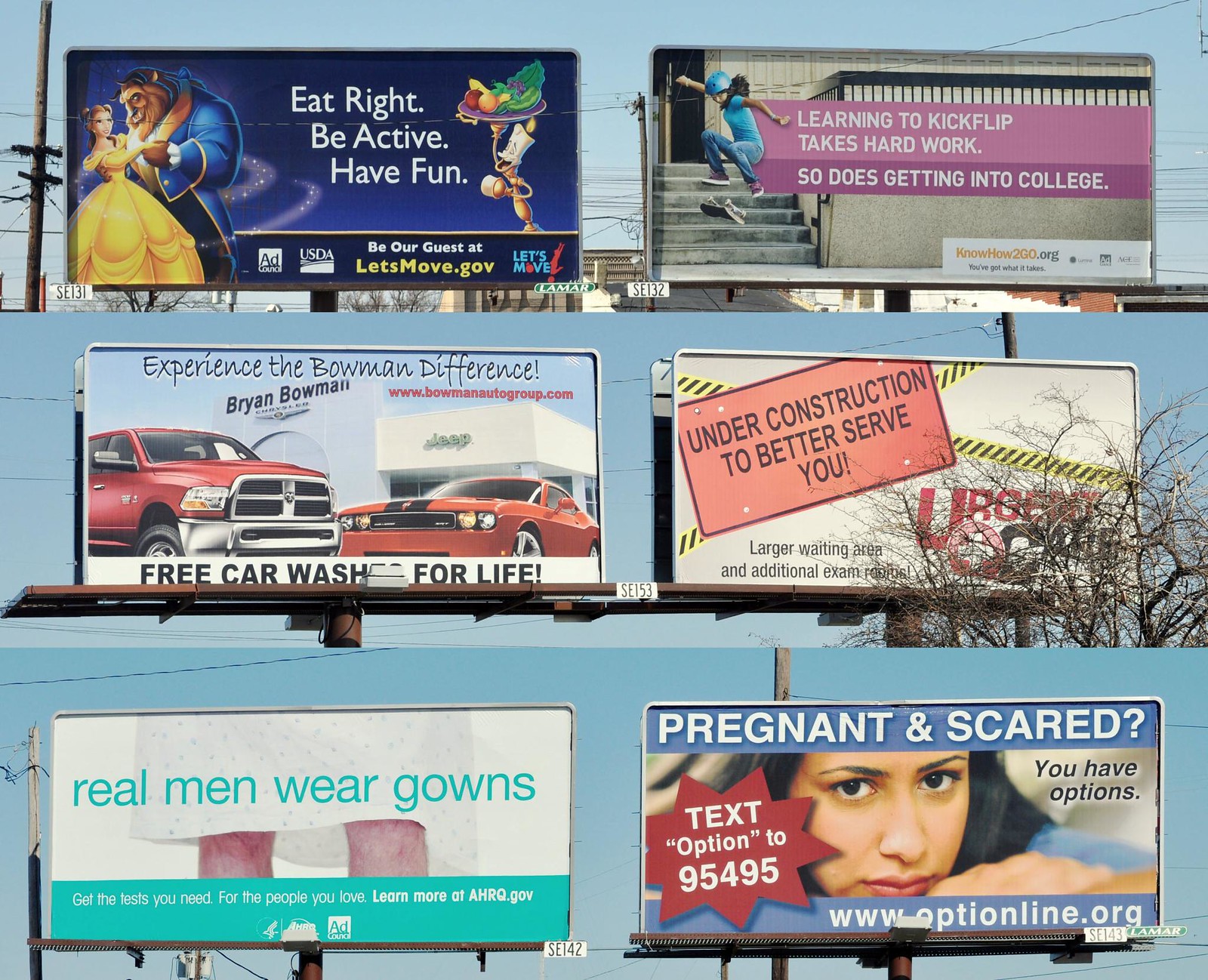A meticulously arranged collage features three rows of panoramic photographs showcasing a variety of billboards from left to right and top to bottom. In the upper left, a vibrant advertisement for "Beauty and the Beast" stands out beside a health-inspired message that reads, "Eat Right, Be Active, Have Fun." The upper right highlights a motivational ad stating, "Learning to Kickflip Takes Hard Work, So Does Getting Into College," encouraging perseverance in both skating and academics.

In the middle row, situated on the left, is a dynamic car and Jeep advertisement with the slogan, "Experience the Bowman Difference." Adjacent to it, a cautionary billboard emphasizes community development with the phrase, "Under Construction to Serve You Better."

The bottom row captures the attention with two impactful messages: On the left, "Real Men Wear Gowns" promotes health consciousness among men; while on the right, a compassionate billboard reassures, "Pregnant and Scared? You Have Options," offering support and resources for those in need.

This detailed display of billboards not only highlights diverse advertising strategies but also reflects a wide range of social, health, and lifestyle themes.